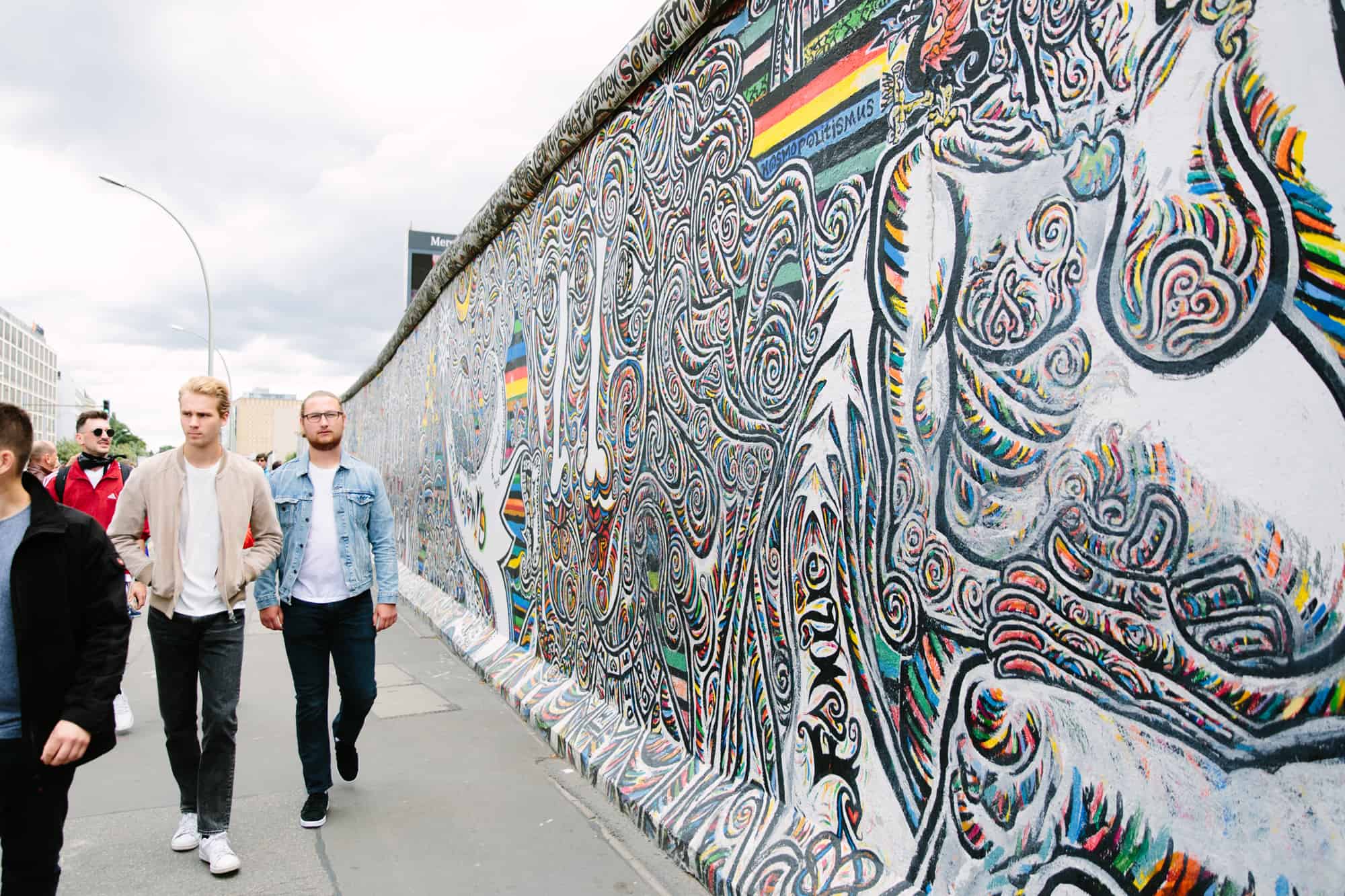This is a horizontally aligned rectangular photograph taken outside on a cloudy day, with the sky visible in the upper left corner covered by white and gray clouds. The image features a group of people walking on a sidewalk. In the foreground, there are two men. The man on the left is wearing a tan hoodie, a white t-shirt, jeans, and white tennis shoes. He has short blonde hair and keeps his hands in his pockets while looking to his right. The man next to him is dressed in a denim jacket over a white t-shirt, black pants, and black tennis shoes. He has small glasses, a shaved head with thin facial hair, and is looking directly at the camera.

The men are walking beside a large, colorful graffiti wall adorned with hand-painted abstract designs that include twirly patterns, circles, stars, arrows, and possibly a bone. The vibrant mural features a spectrum of colors, including red, yellow, blue, purple, pink, black, and white. There is some illegible writing on the wall that might spell "Paul" or "Paulie." Additional people can be seen walking behind the two men in the foreground. Along the sidewalk, there are lamps that line the path, highlighting the lively scene against the backdrop of the expansive, eye-catching mural.